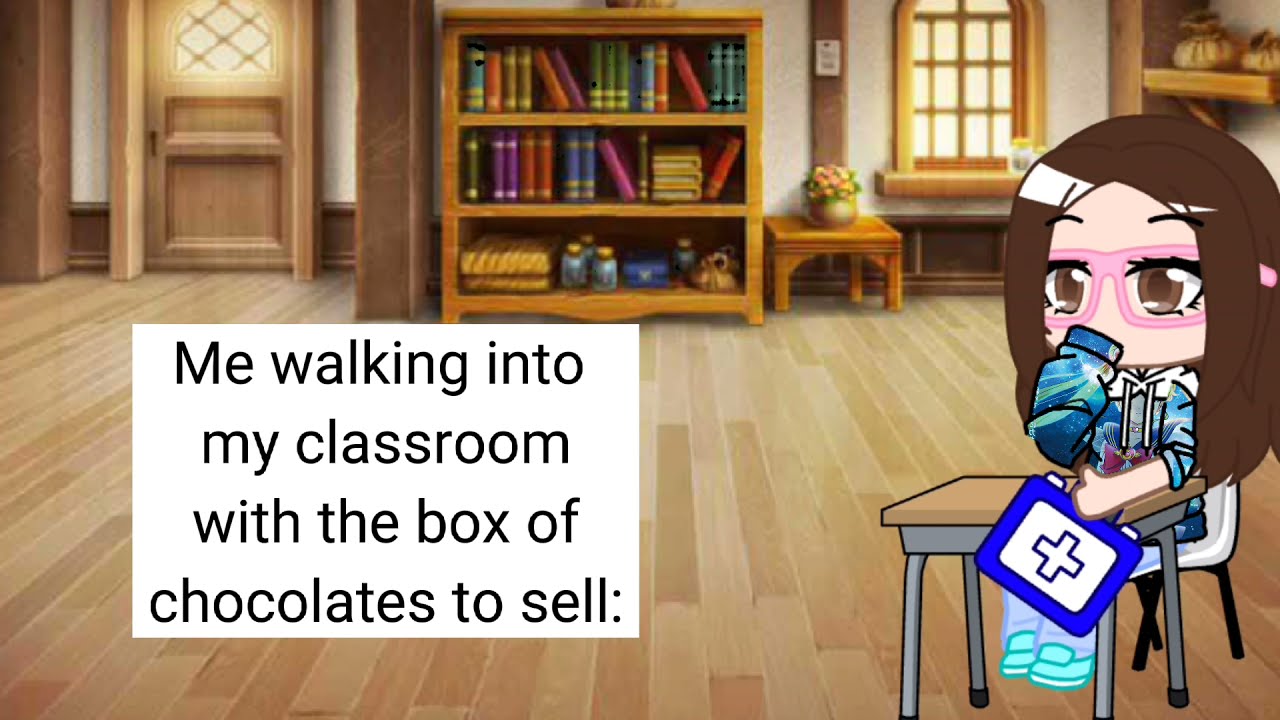The image is a cartoon-style depiction of a school classroom, not rectangular in shape. The classroom features a wooden floor and a white wall. Upon entering the scene, there's a wooden door with a glass window and lattice work on its upper part to the left. In the center of the back wall stands a three-shelved bookcase filled with various books, jars, and boxes. To the right of the bookcase is a small wooden end table adorned with a potted plant with yellow and orange flowers, positioned beneath a window with multiple panes and a thick window sill. Light streams through this wooden-framed window, illuminating the room.

In the foreground on the right side sits a young girl with long, dark brown hair and big brown eyes. She is wearing orange eyeglasses and a blue-green patterned outfit, resembling a tie-dye sweatshirt. Seated at a small desk with a white chair, she holds a blue first aid kit marked with a white cross. Her feet do not touch the wooden floor. The image has a whimsical and stylized appearance, adding to its playful nature.

On the left side of the image, a white sign with black, straightforward printing reads: "Me walking into my classroom with a box of chocolates to sell." Despite the text, the girl is depicted holding a first aid kit instead of chocolates, adding a humorous contrast to the scene.